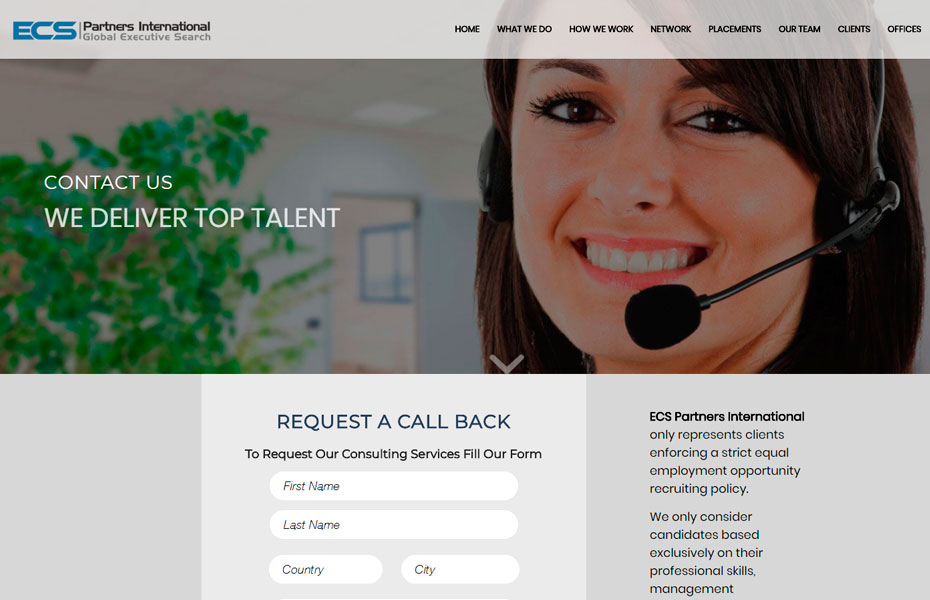This image is a cropped screenshot of a web page belonging to ECS Partners International, showcasing their global executive search services. At the top, prominently displayed, is the ECS Partners International logo. Adjacent to the logo on the right side are the website navigation categories, listed as: Home, What We Do, How We Work, Network, Placements, Our Team, Clients, and Offices.

Dominating the background is a large, high-quality photo of a woman wearing a headset and smiling, symbolizing customer support and approachability. To the left of this image, there's a text overlay stating, "Contact Us - We Deliver Top Talent."

Below the image, the page transitions into a large gray area that constitutes the rest of the webpage's design. At the bottom center of the image, inside a light gray box, there's a clickable button labeled "Request a Call Back." Beneath this button, there's an instruction reading, "To request our consulting services, fill out our form."

The form itself features input lines for "First Name" and "Last Name," followed by "Country" and "City." Flanking this form to the right is a vertically aligned paragraph providing additional information about the company’s services and commitments.